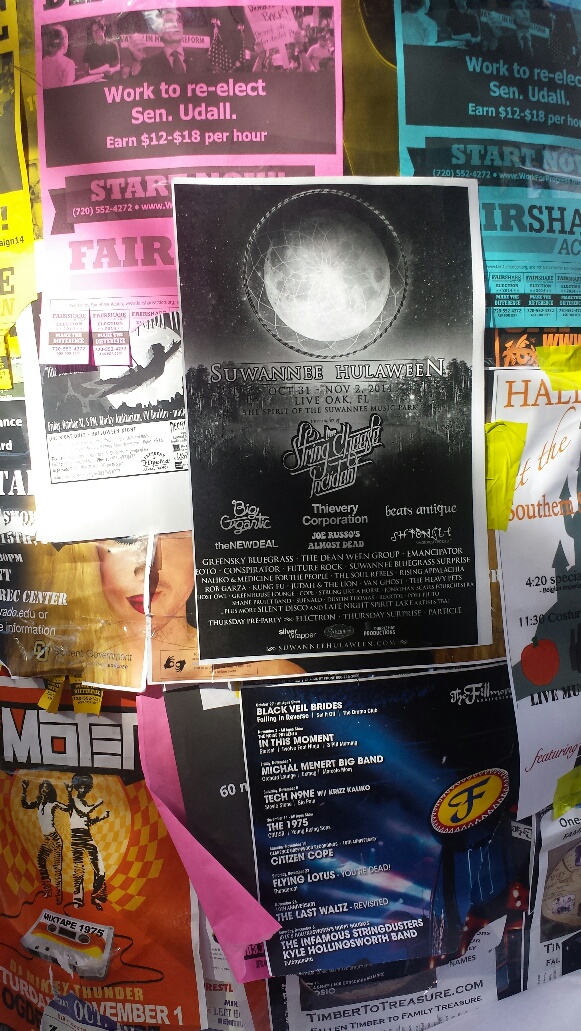The image shows a bustling bulletin board or outdoor pole thick with overlapping, colorful flyers advertising a variety of events and opportunities. Dominating the center is a black and white flyer announcing "Suwannee Halloween" from October 31st to November 2nd, 2014, in Live Oak, Florida, featuring performances by The String Cheese Incident and Big Gigantic. Surrounding this central piece, a mix of papers in white, blue, pink, and yellow offers an array of messages. On the lower left, there's a distinct image featuring people singing and performing adjacent to a cassette tape, hinting at a musical theme. Towards the middle right, a blue flyer lists what appears to be song titles. Noteworthy, in the upper right corner, a blue flyer advertises a job offer with the enticing phrase "Start Now!" promising earnings of $12 to $18 per hour. Scattered throughout are additional flyers obscured by overlap, with some clear details such as "Work to re-elect Senator Udall," a bold yellow and black flyer at the top left, and another for live music events symbolized by motifs like a pumpkin and a moon. These rich, overlapping layers of text and imagery create a vibrant mosaic of community and cultural life.